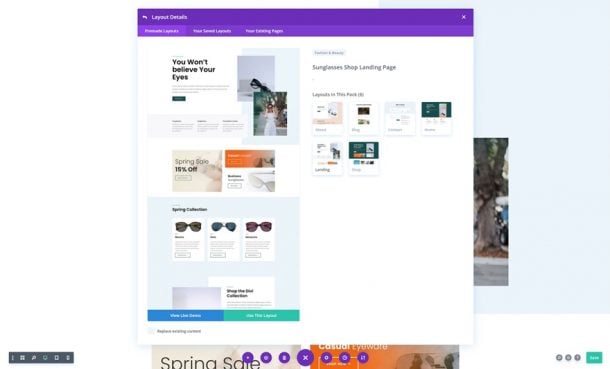In this image, we see a colorful and detailed landing page for a sunglasses shop. In the top left corner, there are layout details for the page design. Prominently in the center, a bold and enticing text reads, "You won't believe your eyes," drawing attention to the striking visuals. Directly beneath this text, a selection of sunglasses is showcased, each positioned to catch the eye of potential customers. 

To the right, a title clearly states that this is the "Sunglasses Shop Landing Page," highlighting the primary purpose of the image. Underneath this title, a brief mention of "Layouts in this pack" suggests that this design is part of a larger collection of templates. Lower on the page, another heading announces the "Spring Collection," accompanied by three distinct sunglasses displayed in black, blue, and brown colors, symbolizing a diverse range within the collection.

The entire page features a vibrant palette including orange, brown, black, purple, green, and blue elements, all set against a clean white background. This combination of colors not only makes the page visually appealing but also enhances the various products being highlighted.